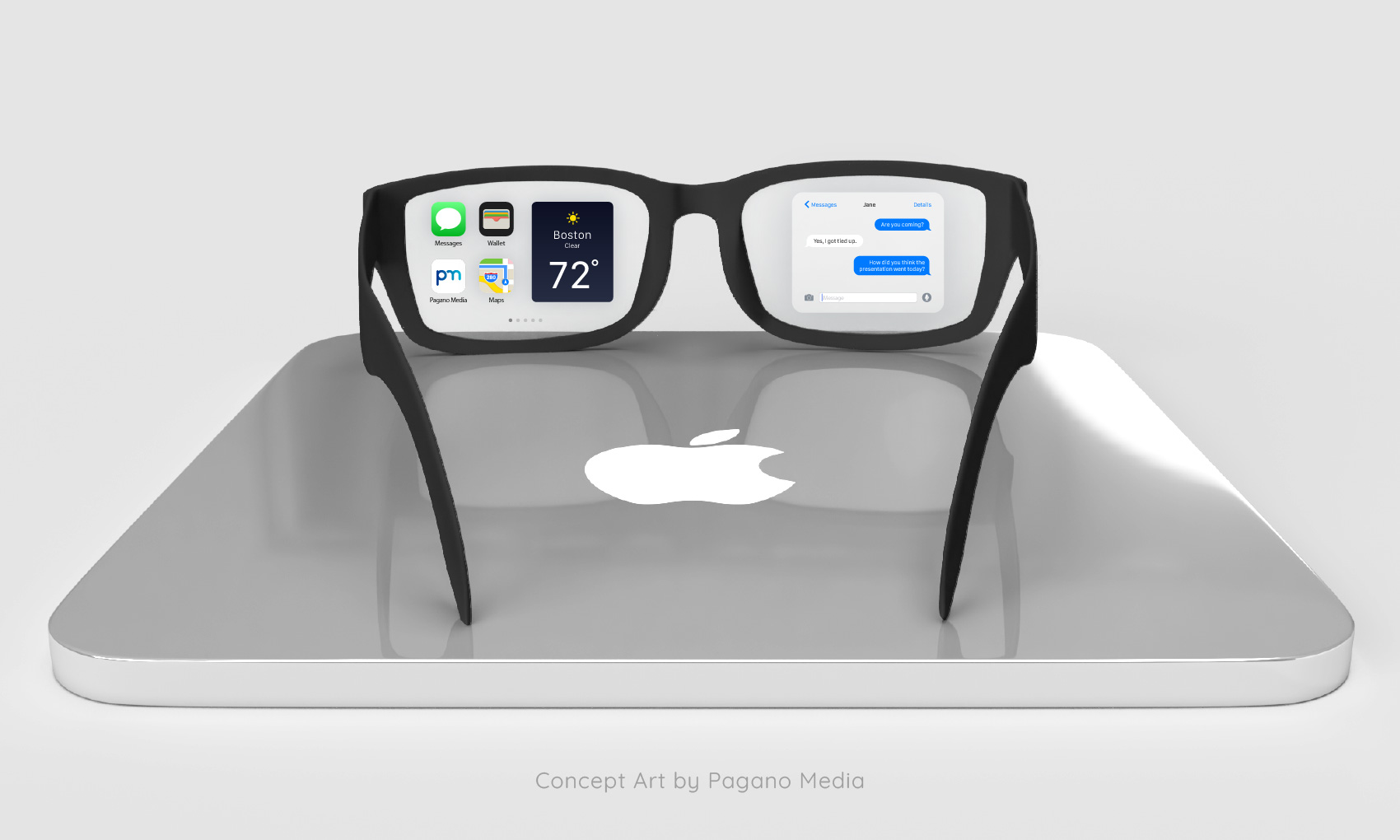This detailed image showcases concept art by Pagano Media, presented with a light gray background. It features a horizontally oriented, silver MacBook or iPad, displayed at an angle with the iconic white Apple logo visible and slightly compressed due to the perspective. Atop this device, a pair of black-framed glasses are prominently placed, with their earpieces oriented towards the camera.

The glasses appear to be an advanced virtual or smart eyewear concept, offering augmented display capabilities. The left lens features various widgets, including a weather update indicating '72 degrees in Boston' within a black square, a messages app (with green and white text bubbles), and additional icons for Wallet and Maps apps. The right lens shows an active chat interface with yellow and white text bubbles, suggestive of ongoing communication.

The entire scene is subtly branded at the bottom with "Concept Art by Pagano Media," seamlessly blending innovative design and digital functionality, emulating an immersive, futuristic Apple advertisement.